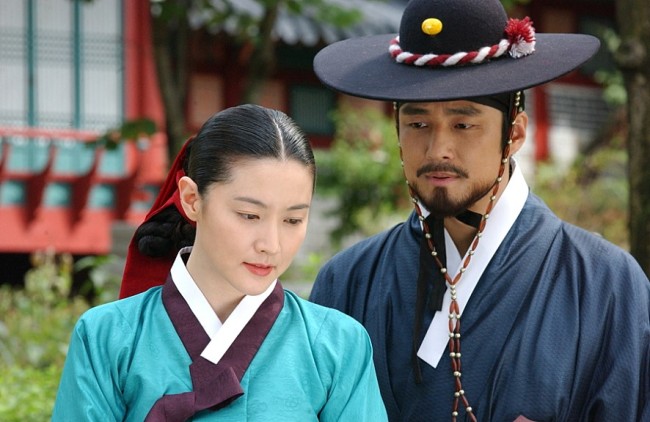In this outdoor photograph, an Asian man and woman are standing side by side, with the man positioned slightly behind the woman. The woman, who has black hair adorned with a red accessory at the back, is looking downwards and is dressed in a light blue, robe-like garment featuring purple and white collars. The man, taller than the woman, is gazing at her. He is wearing a navy blue robe with a white collar and a brimmed black hat decorated with a yellow detail on the front and a red-and-white twisted rope around it, which also serves as a chin strap. The background is somewhat blurred but reveals a couple of trees, bushes, and an orange-colored building with green window frames. The overall scene is set in a landscape orientation, with no other people present in the image and no text or numbers visible. The color scheme prominently includes black, red, white, yellow, purple, and blue tones.